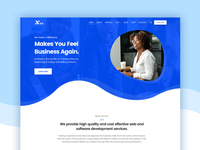The image depicts a computer screen displaying a webpage with a predominantly light blue background at the top, transitioning into royal blue with gentle, wavy curves separating it from a white area below. At the top, barely visible but perceptible, are three individuals standing, seemingly engaged in a discussion or a task, possibly looking down at something on a table. The phrase "Makes you feel business, makes you feel business again" is prominently displayed, capturing attention at the top of the page. Due to the blurriness, a sentence in the white area and some smaller text below it are indiscernible, though their presence hints at additional content.